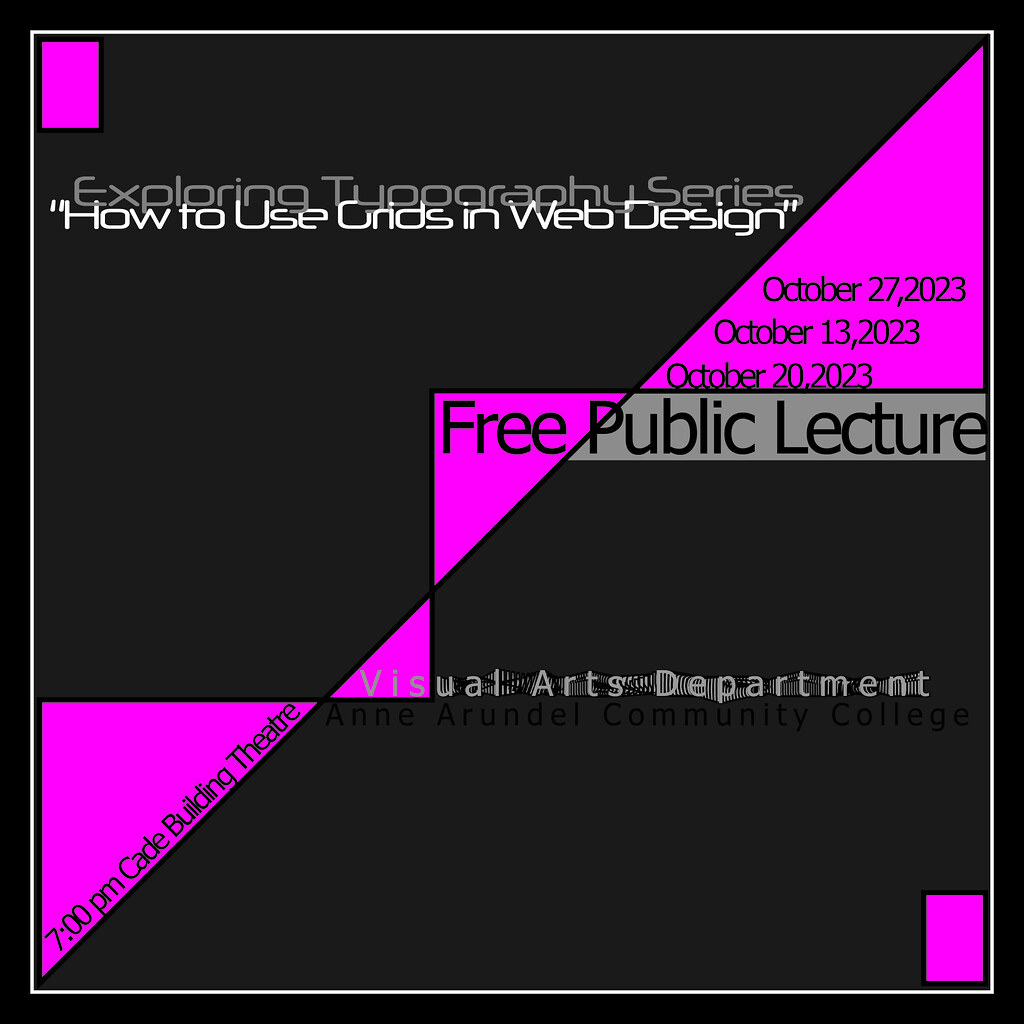This is an advertisement for a public lecture featuring a geometrically designed image with a grey square background accented by various pink triangles of different shapes and sizes on each side. A vertically positioned pink rectangle adorns the top left corner. The ad is bordered by a thin white outline with a darker grey backdrop extending outside the border. The main text, written in white and grey, promotes the "Exploring Typography Series" under the title "How to Use Grids in Web Design." Additionally, within one of the pink triangles, the dates October 13, 2023, October 20, 2023, and October 27, 2023, are listed. The lecture is a free public event hosted by the Visual Arts Department of Anne Arundel Community College, held at 7 p.m. in the Cade Building Theater.